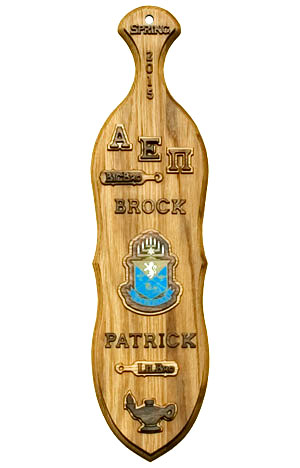In the center of the image, there is a wooden paddle with a stained light brown finish, displayed against a stark white background, giving it a floating appearance. The paddle is oriented with the handle at the top and the broader end at the bottom. Carved prominently at the top is the word "Spring," followed by the year "2015" arranged vertically below it. A set of Greek letters, reading "ΑΕΠ" (Alpha Epsilon Pi), is inscribed beneath the year. Further down the paddle, there's a depiction of an object that could be interpreted as a beer bottle or telescope. The name "Brock" is etched next to this image. Lower on the paddle, there's a blue shield, possibly accompanied by what appears to be candles and the name "Patrick" inscribed. At the very bottom of the paddle, there is an illustration of a genie lamp. The predominantly brown paddle is accented with shades of greenish-gray, blue, dark brownish-black, and white, contributing to its detailed design.